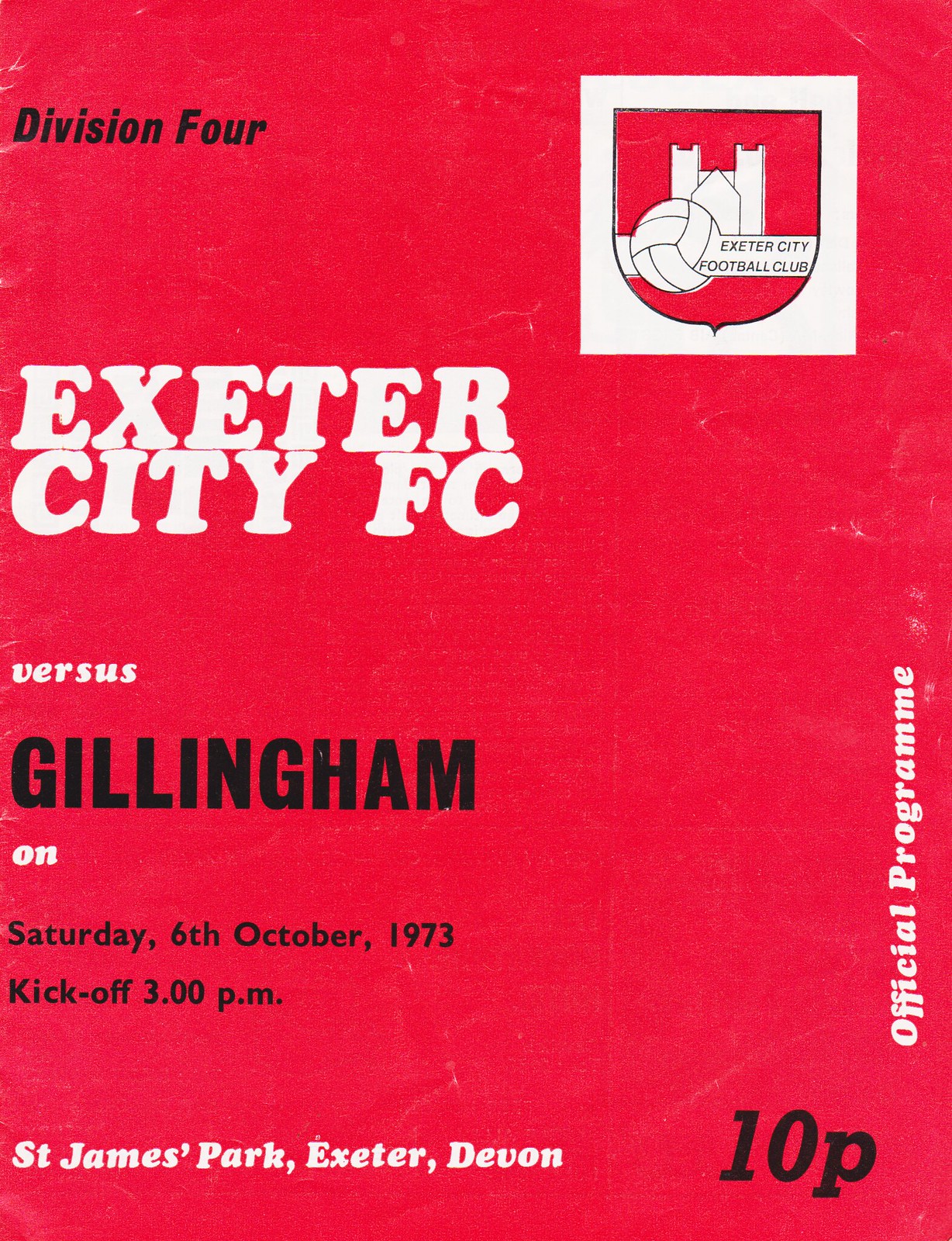The image is a magazine or sports program cover with a solid red background. In the top left corner, black text reads "Division 4," and below it, in bold white text, is "Exeter City FC." The text continues with "Versus Gillingham" in black. The date of the event, "Saturday, 6th October 1973," and the time, "Kickoff 3pm," are also in white text on a black background. A notable feature in the top right corner is a red shield emblem with a white border, illustrating a football and a building, labeled "Exeter City Football Club." The bottom left corner specifies the venue as "St. James Park Exeter Devon." In the bottom right corner, a black number and letter read "10P," indicating the price. Running vertically along the right side in white text is the label "Official Program."